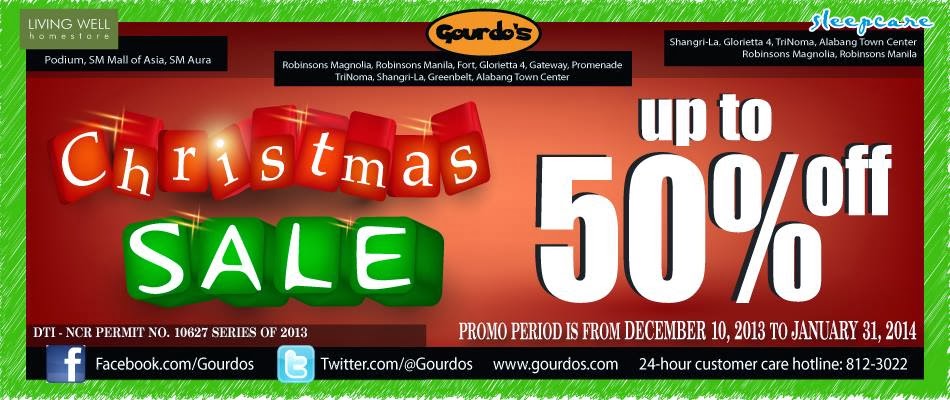The image features a detailed promotional banner from the Livingwell Home Store. The top-left corner prominently displays the store's name, "Livingwell Home Store," against a dark green background. The interior of the banner is primarily red, framed by a green border adorned with diagonal scribble designs that add a playful touch.

At the top center of the image, there's an eye-catching orange oval with the word "Gourdos" (spelled "G-O-U-R-D-O-S") featured in white lettering. To the right of this oval, the words "Sleep Care" are displayed.

Beneath the "Livingwell Home Store" title, additional text reads: "Podium 5M, All of Asia, SM Aura." Below the "Gourdos" oval, a list of locations is provided, including: "Robinson Magnolia, Robinson Manila, Fort Granada, The Gateway, Promenade, Trinoma, Shangri-La, Greenbelt, Alabang Town Center." 

On the right side of the banner, listed vertically, are the following locations: "Shangri-La, Glorietta, Alabang Town Center, Robinson Magnolia, Robinson Manila."

A promotional message at the bottom right corner announces a "Christmas Sale" with discounts of up to 50% off.